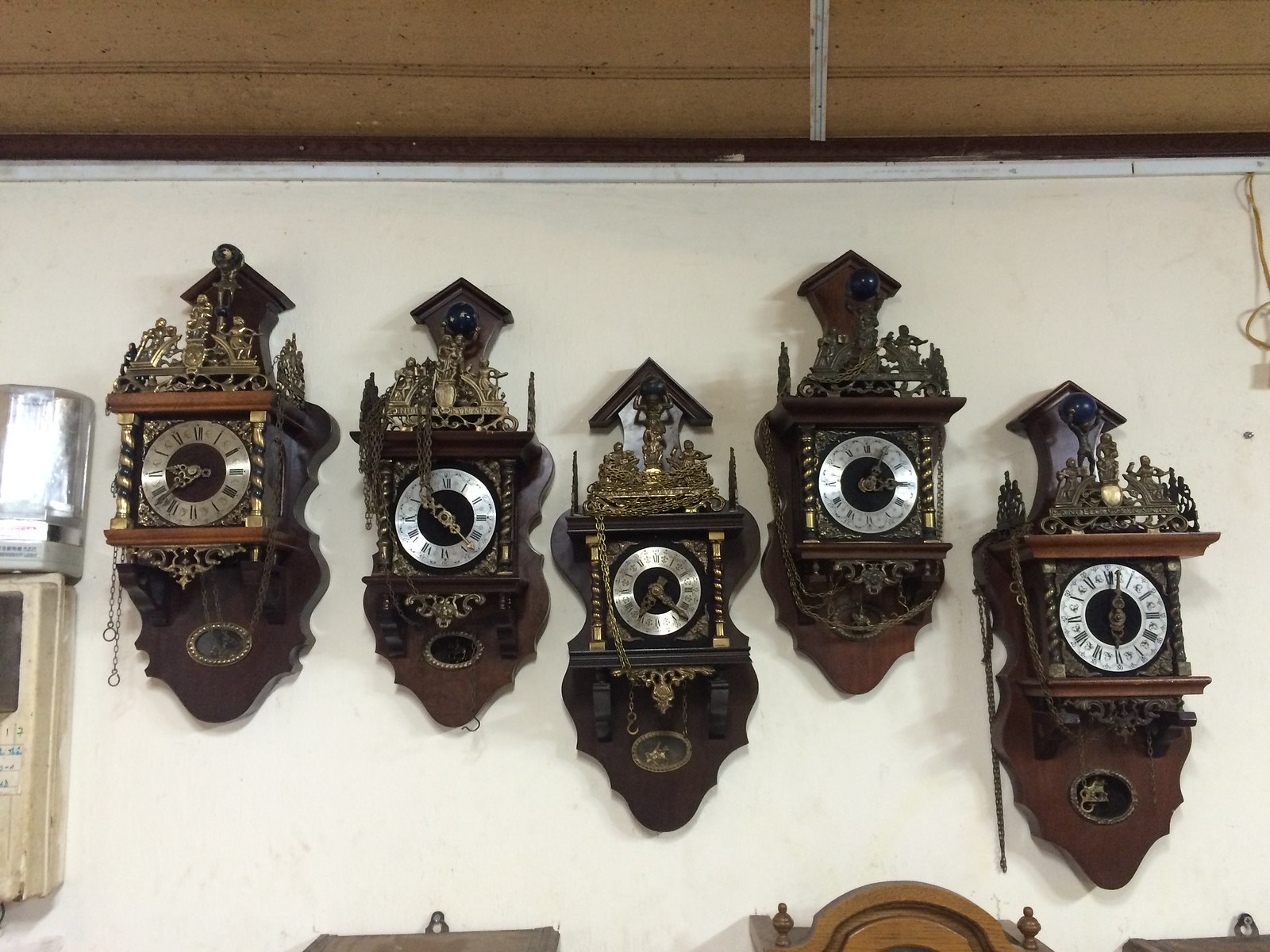The image showcases a series of five ornate, antique cuckoo clocks mounted on a somewhat aged, cream-colored wall, reflective of an old building. Each of these meticulously crafted clocks is predominantly wooden, varying in shades from dark brown to milk chocolate. They exhibit elaborate decorative elements, such as gold and brass embellishments, including statues and ornamental figures often positioned at the top. The clock faces are predominantly silver, featuring black numerals and a mix of gold and silver hands. Some clocks have additional decorations like gold columns flanking the sides of the dials. The overall arrangement shows the clocks almost aligned, with one or two positioned slightly lower than the others. At the bottom edge of the image, parts of three smaller clocks are visible. The wall's aged condition, with portions of worn paint, underscores the vintage charm of the display.